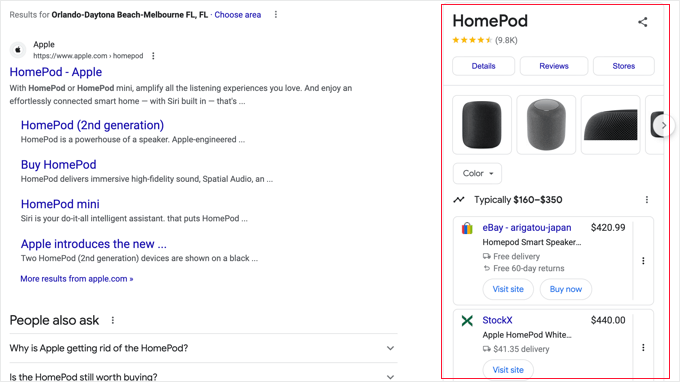The image showcases a search results page for various locations in Florida, including Orlando, Daytona Beach, and Melbourne. Just below these listings is a highlighted blue option to choose the area, which is a clickable link. The website for Apple is featured, alongside an Apple logo and the URL "https://www.apple.com/homepod".

Highlighted in bold blue are the words "HomePod - Apple". Below this, in black font, it reads: "With HomePod and HomePod mini, amplify all the listening experiences you love and enjoy an effortlessly connected smart home with Siri built-in." This is followed by an ellipsis.

Next, in dark blue text, it says "HomePod (2nd generation)" within parentheses. Underneath, it states in black: "HomePod is a powerhouse of a speaker Apple engineered." Then in bold blue, it says "Buy HomePod." The black text underneath reads: "HomePod delivers immersive high-fidelity sound, spatial audio, and..." followed by more text cut off by ellipses.

Further details highlighted in bold blue read "HomePod mini," and underneath it states in black: "Siri is your do-it-all intelligent assistant that puts HomePod...". Additionally, there's a heading in bold blue stating "Apple introduces the new..." followed by "HomePod" in black font. Two HomePod (2nd generation) devices are shown in the image.

Below these results are the words "More results from Apple.com," leading into readily visible FAQs under "People also ask". The two questions listed are: "Why is Apple getting rid of the HomePod?" and "Is the HomePod still worth buying?" each with a down-arrow for expanding the answers.

To the right of the photo, several HomePod versions are displayed, including details, reviews (currently 9.8k reviews), in-store availability, a color filter option, and a price range of $160 to $350. Additionally, an eBay user named "Ligatou-Japan" offers a HomePod smart speaker for $420.99 with free delivery and 60-day returns, alongside buttons to visit the site or buy now.

Another seller, StockX (not eBay), lists the Apple HomePod (white) for $440.00 with a delivery fee of $41.35. There is also a button to visit this site.